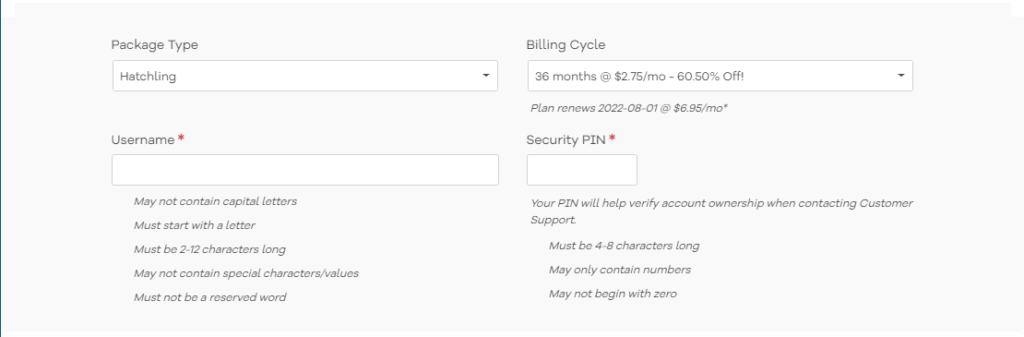The image displays a web page form with a subtle, nearly transparent design that makes it easy to overlook at first glance. The background is white, and the text is in an extremely faint blue font. The most prominent feature is a long blue line that runs vertically along the left-hand side of the page, providing definition amidst the otherwise soft visual elements. 

The page contains information about a subscription package. It specifies that the package type is "Hatchling," with a billing cycle of 36 months at a rate of $2.75 per month, offering a substantial discount of up to 50%. It notes that the plan will renew on January 1, 2028, at a rate of $6.95 per month.

Additional fields include sections for entering a username and a security PIN, each accompanied by corresponding input boxes. The username field has specific requirements: it must be 2 to 12 characters long, start with a letter, and should not contain capital letters. Further instructions and constraints for these fields are provided, adding clarity to the form-filling process.